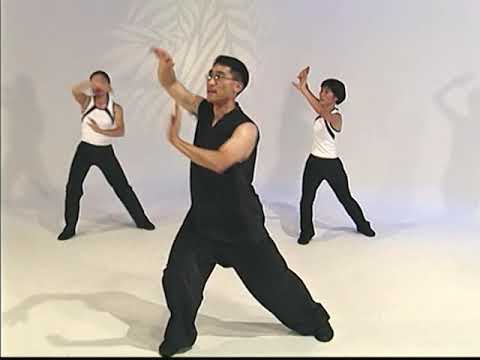The image appears to be a low-resolution still from a Tai Chi instructional video. In the foreground, a man in his late 30s, wearing a sleeveless black martial arts gi and baggy black pants, is performing broad, Tai Chi-like gestures. He has glasses and is positioned with his right arm raised to about forehead level, palm facing out, and his left arm extended in front of him also with the palm out. His stance shows his left leg extended back as he bends forward on his right leg. Flanking him are two young women, mirroring his movements. Both wear white sleeveless tops with black stripes, paired with black loose-fitting pants and black shoes. The background is predominantly white, illuminated by multiple light sources casting various shadows, and decorated with a projected floral pattern that adds a touch of color and texture. All three individuals are engaged in synchronized Tai Chi movements, emphasizing the instructional nature of the scene.